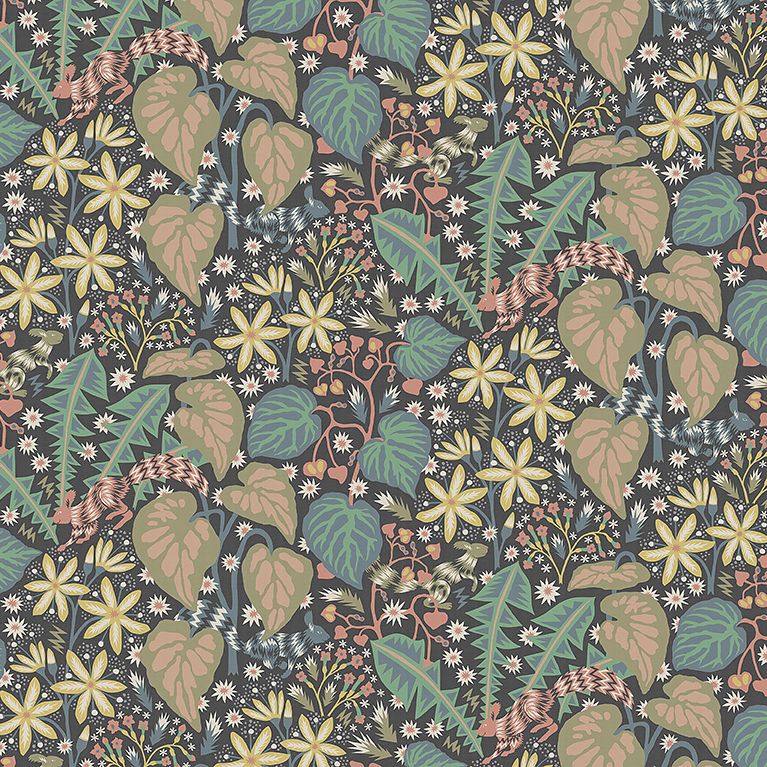This image showcases a contemporary Scandinavian-style digital design featuring a meticulously detailed repeating pattern. The motif predominantly includes floral and woodsy elements, such as a variety of green leaves, including ivy. Central to the design are vibrant yellow daisies, complemented by tiny pink flowers scattered throughout. Subtle, muted hues give the pattern a harmonious balance. As one examines the image closer, small, whimsical squirrels become visible, adding a charming touch. Despite the dense array of elements, with minimal background space, the design maintains a high level of aesthetic cohesion, creating an overall captivating and intricate piece of work.